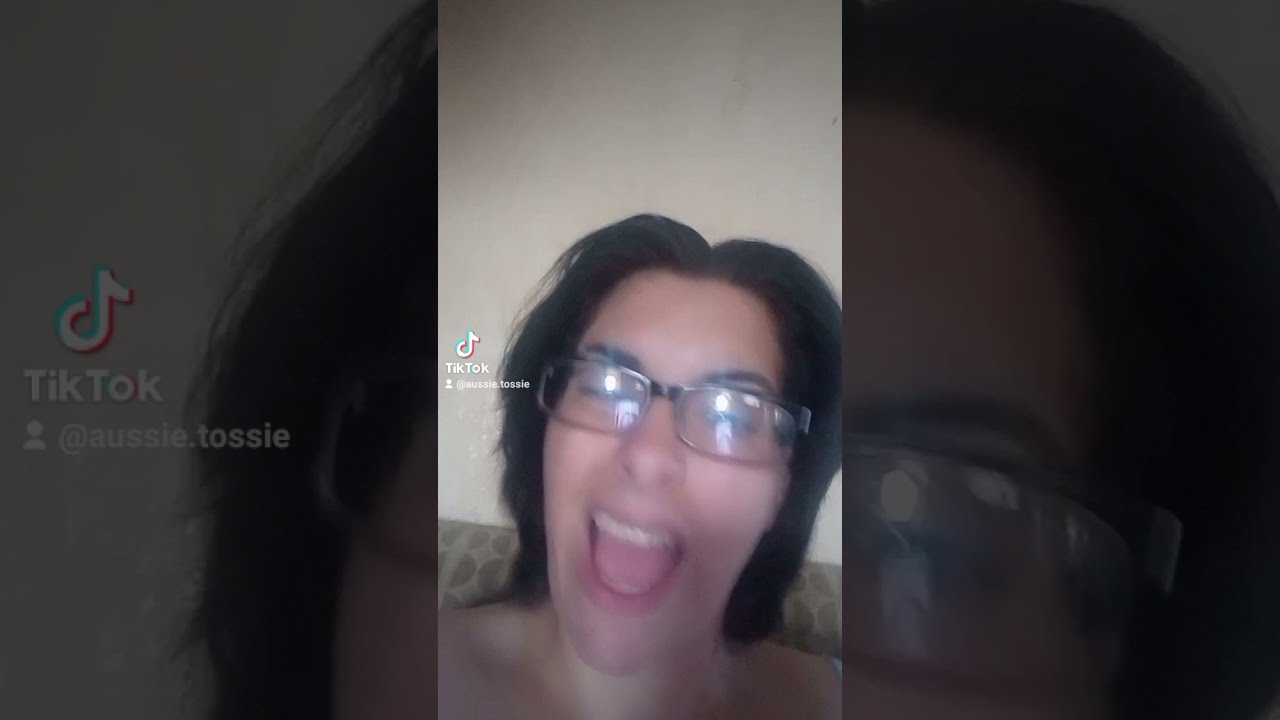In this detailed image, a still from a TikTok video showcases a woman, assumed to be the user @ozzy.tozzy, sitting on a tan, fabric couch with a subtle polka dot pattern. The woman, framed from her collarbones upward, is positioned centrally with the TikTok logo and her handle situated to the left of her face. Her shoulder-length, dark hair frames her face as she appears to be either yelling or singing, with her mouth wide open exposing a pink tongue and top teeth. Her thick eyebrows are prominent above slightly closed eyes, and she is wearing silver-framed glasses that reflect the light in the room. The background features a plain white wall, providing contrast to the more vivid elements in the foreground.